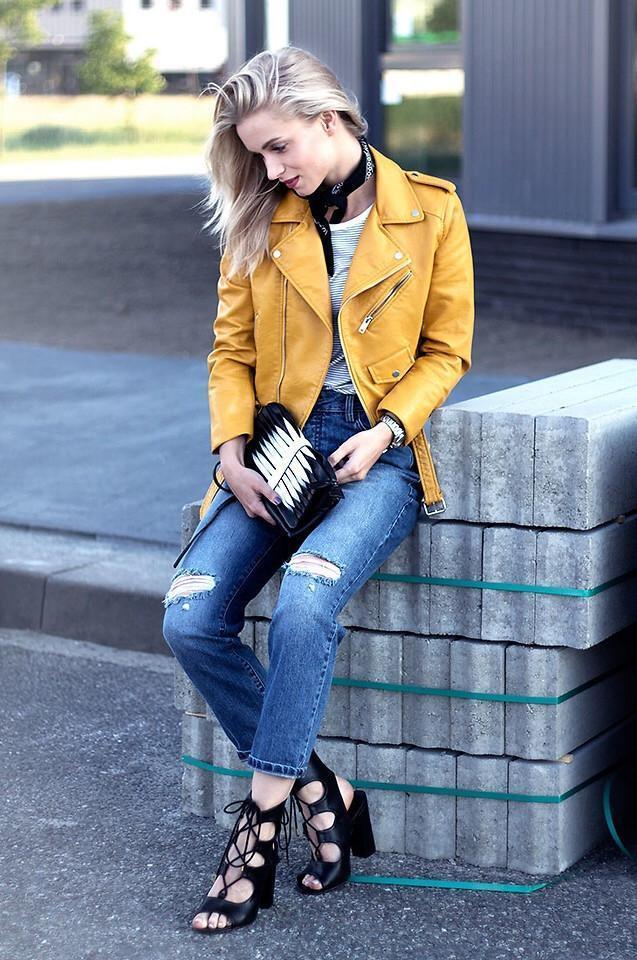The image captures a striking blonde woman in her twenties, sitting on a stack of gray concrete blocks that resemble construction materials. She is dressed in a vibrant yellow leather jacket over a white shirt, paired with ripped blue jeans that reach her ankles. Her footwear includes black, laced-up high-heeled shoes. She carries a small black purse with white stripes. The woman has long, flowing blonde hair, a beautiful face adorned with red lipstick, and a black scarf around her neck. The setting is outdoors on a sidewalk, with a background of trees and part of a building illuminated by daylight.